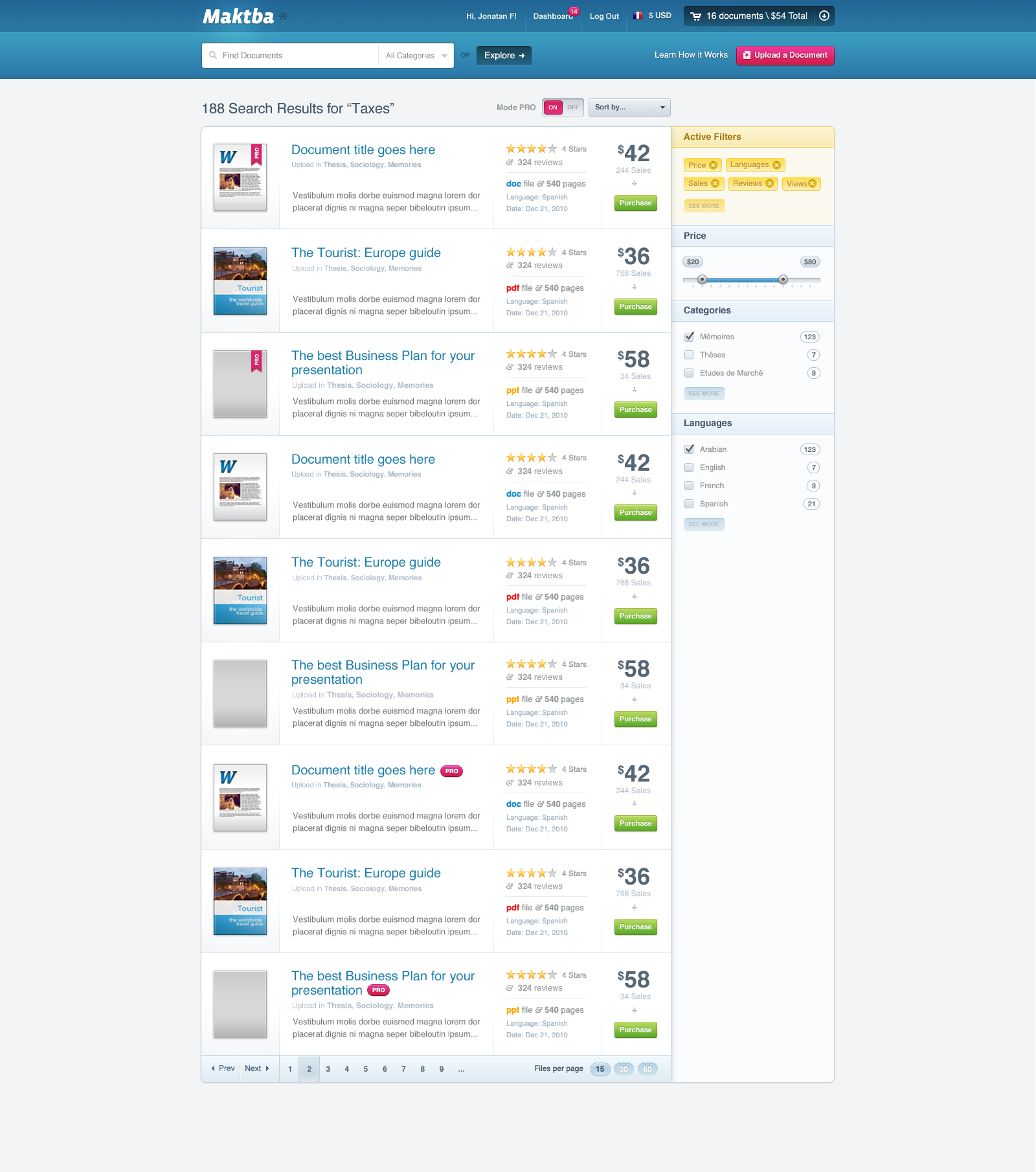The image depicts a webpage from Maktba, which is displayed with a dark blue ribbon across the top. On the left side of the ribbon, "Maktba" is prominently written in bold white text. To the right, smaller white text says "Hi" followed by a user's name (though it's very tiny and difficult to read). Next, the word "Dashboard" appears with a red dot beside it indicating notifications. Following this are links for "Log Out," an currency indicator "USD," and an icon of a shopping cart in gray with a white shopping cart symbol.

Below the ribbon, there's a white search bar centrally located with a black "Explore" button to its right, which has "Explore" written in white. Some smaller text, which is unreadable, is displayed to the right of the button. The section below the search bar reveals the text "188 search results for taxes" set on a very light gray background.

The primary content area features a long vertical white box listing search results related to taxes. Each search result is highlighted in bright blue type, accompanied by a star rating and a price indicator. This structured listing provides a comprehensive overview, making it easy to browse through the various options available.